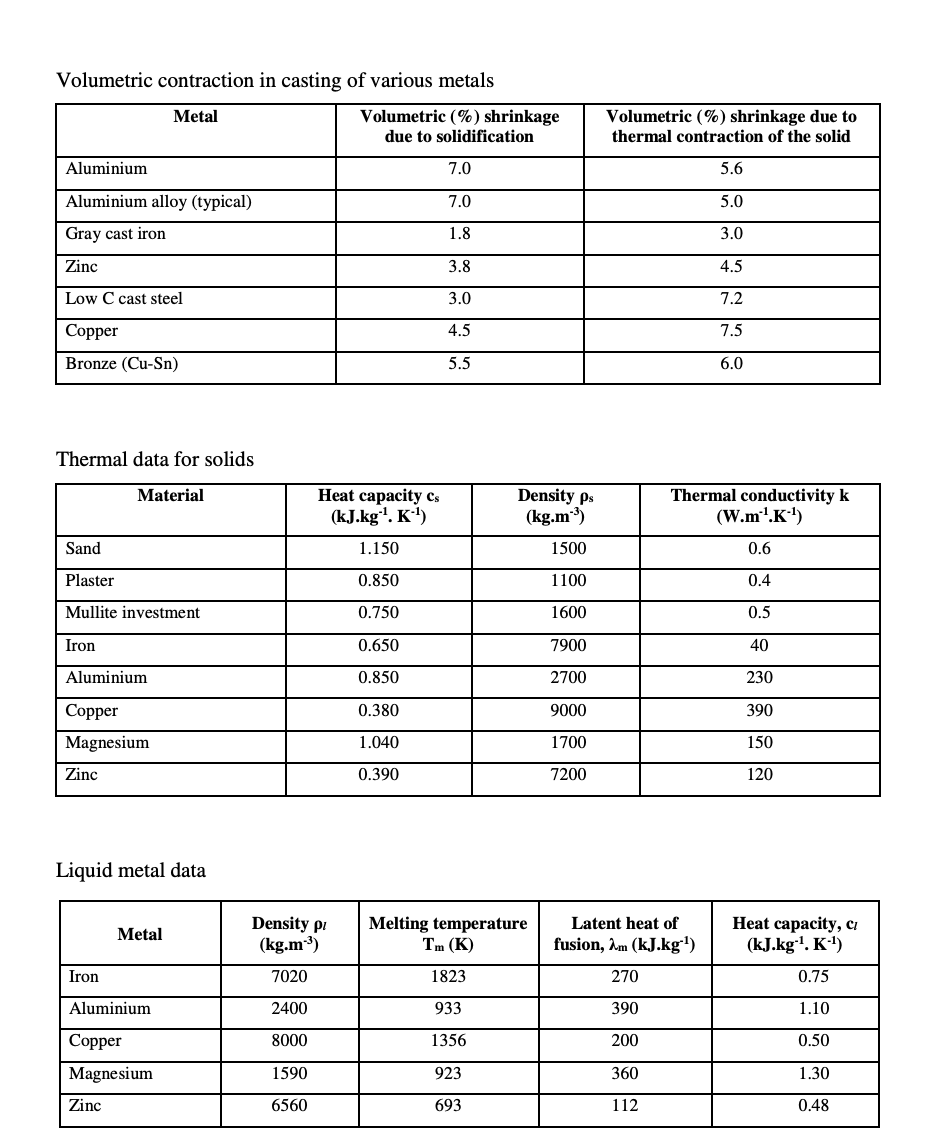The image features three vertically stacked, horizontally rectangular data tables in black and white text. The first table, titled "Volumetric Contraction in Casting of Various Metals," includes three columns: "Metal," "Volumetric Percentage Shrinkage Due to Solidification," and "Volumetric Percentage of Shrinkage Due to Thermal Contraction of the Solid." The metals listed are aluminum, aluminum alloy (typical), gray cast iron, zinc, low C cast steel, copper, and bronze.

The second table, titled "Thermal Data for Solids," presents four columns: "Material," "Heat Capacity," "Density," and "Thermal Conductivity." The materials in this table are sand, plaster, molite investment, iron, aluminum, copper, magnesium, and zinc.

The third table, titled "Liquid Metal Data," encompasses five columns: "Metal," "Density," "Melting Temperature," "Latent Heat of Fusion," and "Heat Capacity." The metals listed are iron, aluminum, copper, magnesium, and zinc.

This comprehensive chart is likely intended for manufacturers or individuals involved in casting various metals, providing essential data on volumetric shrinkage, thermal properties, and melting points.